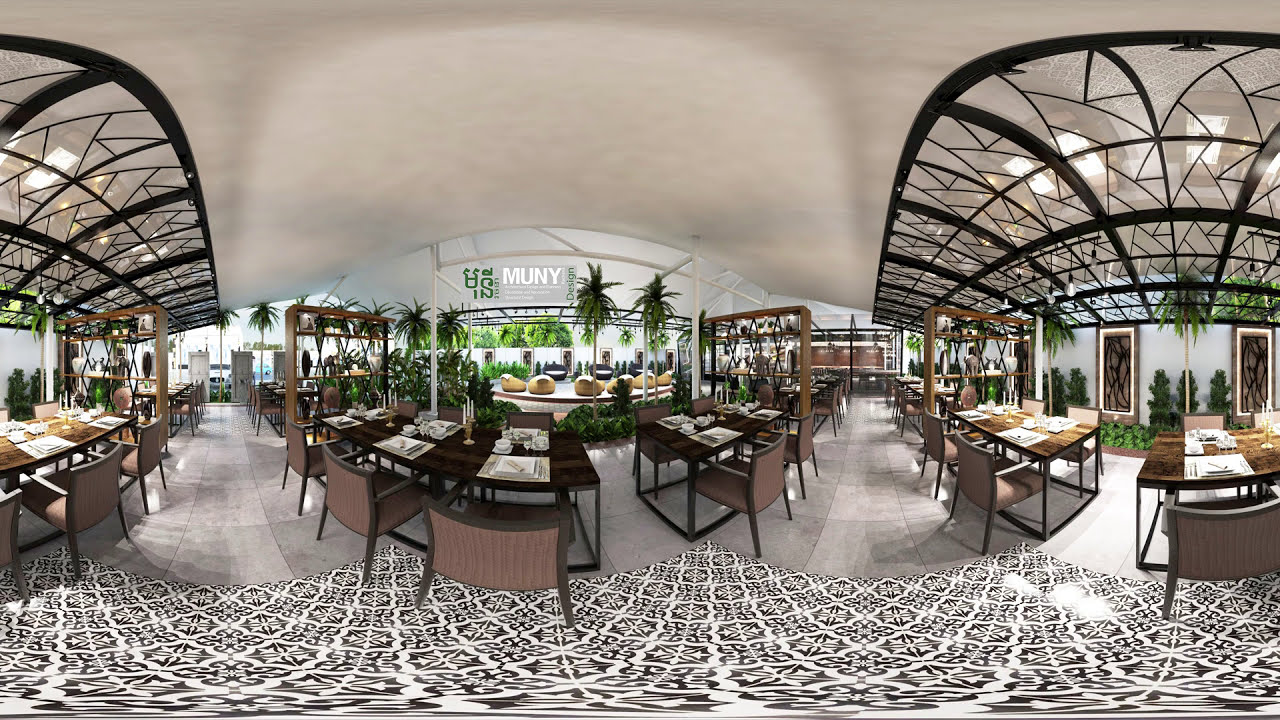The image showcases the interior of a sophisticated restaurant with a slightly warped, 360-degree perspective, giving it a photorealistic yet slightly animated feel. The floor in the foreground of the restaurant features an intricate black and white pattern that transitions into slate-gray stone tiles as it recedes into the background. Dark wood tabletops are elegantly set with white plates and beige placemats, accompanied by gold candelabras topped with white candles. Each table is paired with stylish brown rattan chairs framed in black. 

The ceiling is predominantly white, accented by striking black metal and glass designs. Tables are arranged in a U-shape and separated by large wood dividers adorned with various metals and decorative elements. Lush greenery, including hanging plants and potted trees, adds a touch of nature to the ambiance. 

Near the center of the image, a sign that reads "MUNY" in bold letters hangs above a countertop, suggesting either the name of the establishment or a distinct design feature. Distinctive lighting fixtures framed in black glass panels illuminate the area, enhancing the refined atmosphere. The restaurant appears to be ready to welcome guests but currently sits empty.